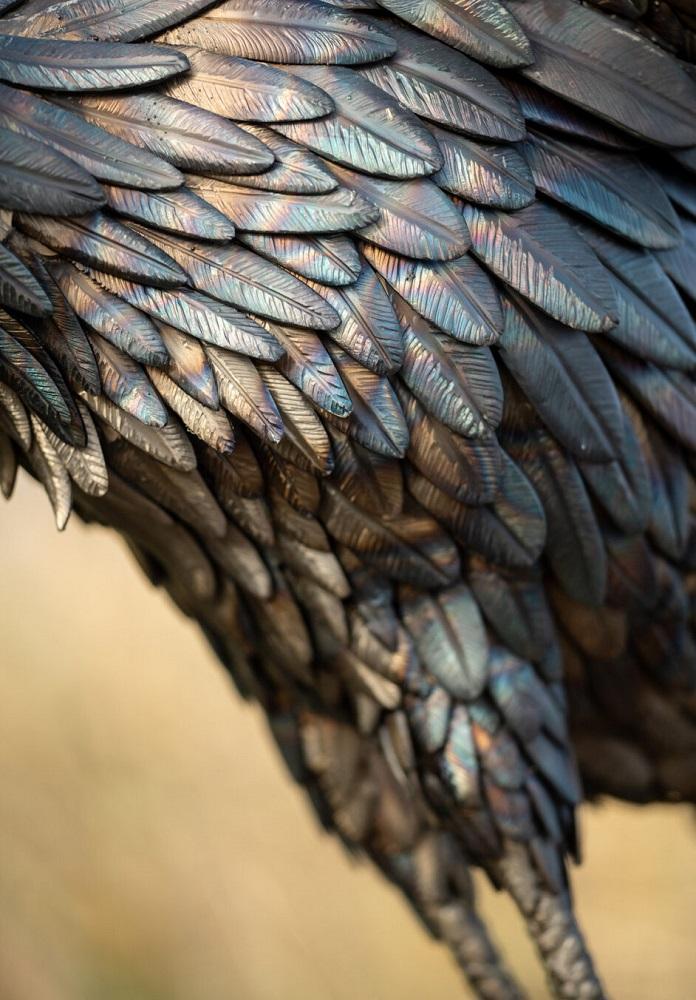This detailed image captures a burnished, metallic sculpture of a bird set against a slightly out-of-focus yellow-beige background. The composition showcases the bird's legs up to the thighs, meticulously depicting the textured scales, yet the feet are omitted. The bird's intricate plumage—ranging from small to large, and oriented symmetrically—dominates the frame, extending from the breast along its side. Each feather, beautifully solid with detailed center quills, exhibits a fascinating spectrum of colors from light brown, pearlescent blue, to near black, creating an almost fired appearance. This piece, resembling perhaps a crow, displays a subtle rainbow-like iridescence across its feathers. Though the wings, head, and tail are not visible, the bird's body is elegantly highlighted, making the viewer appreciate the intense craftsmanship and the artistic representation of its natural form.